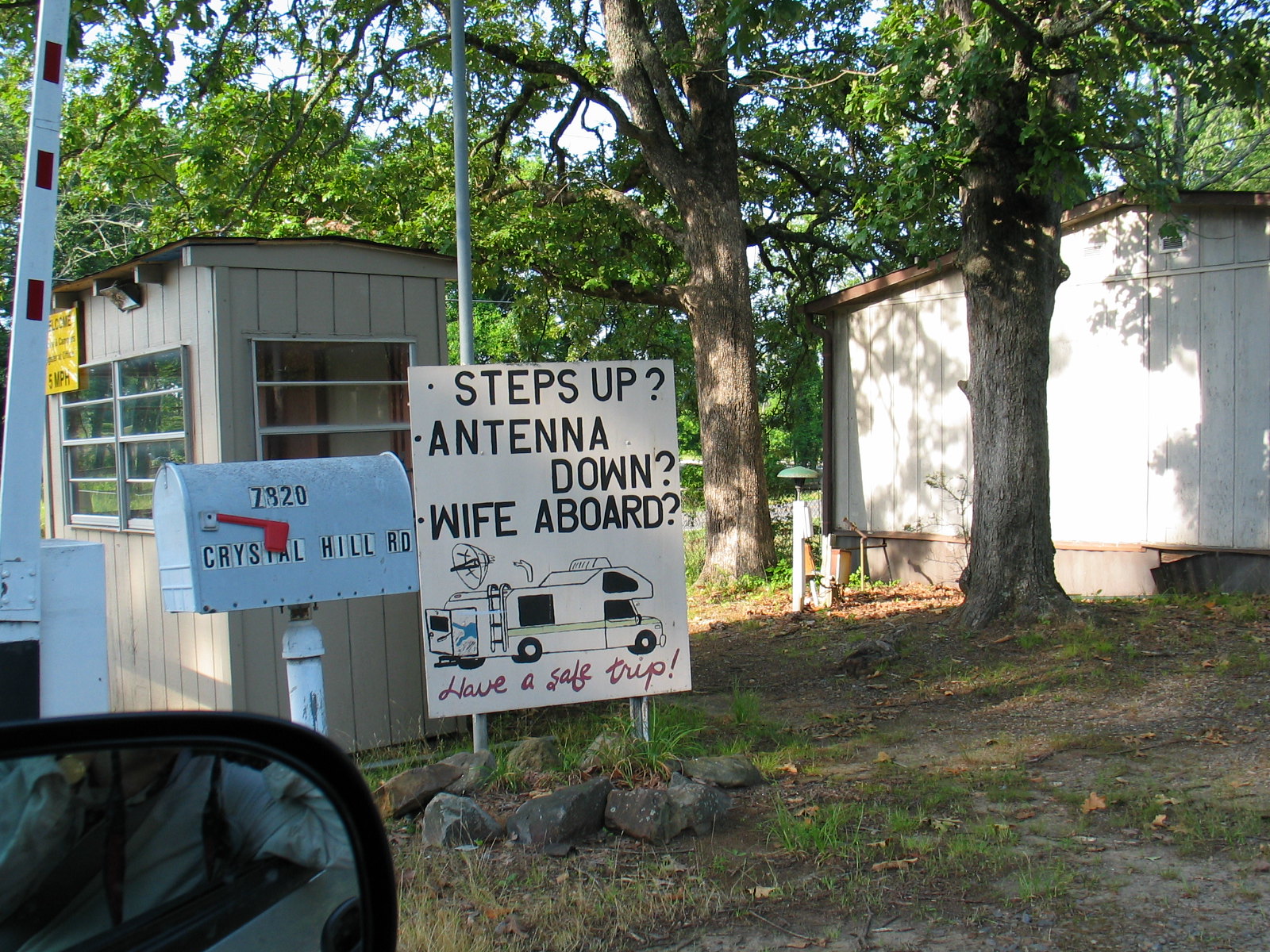The image showcases the entrance to a campground, captured from the passenger side of a car. The lower left-hand corner of the photo reveals the passenger side mirror, reflecting a portion of a person’s neck, left hand, left shoulder, and the sleeve of a gray sweatshirt. Prominently displayed in the middle of the image is a white sign featuring the message, "Steps up, antenna down, wife aboard." Beneath this message, the sign wishes travelers, "Have a safe trip." This detailed scene captures the essence of preparedness and a friendly send-off typical of camping culture.